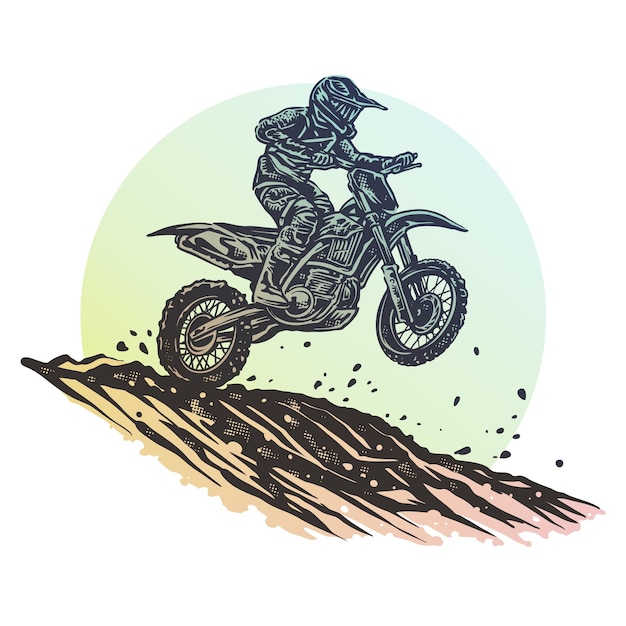The image depicts a stylized, pop art-inspired drawing of a motocross rider performing a wheelie on a dirt bike. The rider is clad in full motocross gear, including gloves and a helmet with a visor, rendered entirely in black with light green accents. The dirt bike's tires, muddied as they carve through the terrain, show the back tire firmly on the ground while the front tire is lifted, capturing the dynamic motion of the stunt.

The background features a prominent, large sun in green and yellow hues, dominating the all-white background. The sun's circle contrasts with the monochrome and subtly colored elements of the artwork. The ground beneath the bike is depicted with a mix of beige, light brown, and polka-dotted black textures, suggesting a rocky, dirt path. Black specks and rocks are illustrated flying around the bottom of the image, emphasizing the ruggedness of the terrain and the action involved.

Overall, this whimsical and energetic graphic, with its carved, stamp-like details and playful color scheme, resembles the type of artwork typically found on a child's t-shirt.